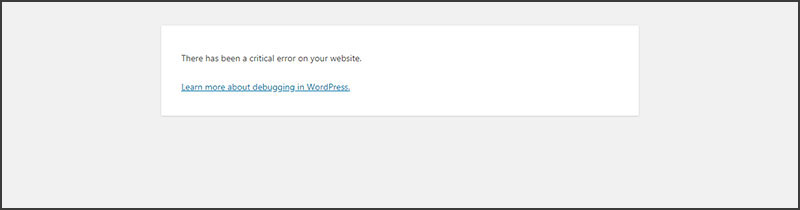The image features a notification displayed prominently in a white rectangular box positioned slightly towards the top center. Inside the rectangle, the message "There has been a critical error on your website" is written in bold black text, alerting the viewer to a significant issue. Directly beneath the error message, a blue hyperlink labeled "Learn more about debugging in WordPress" offers a potential solution by guiding the viewer to further information. The entire notification is set against a light gray background, providing a neutral contrast that emphasizes the message. A thin black border outlines the white rectangle, adding definition and framing the notification within the image. The composition is simple yet effective, focusing solely on conveying the urgent message and its related assistance link.